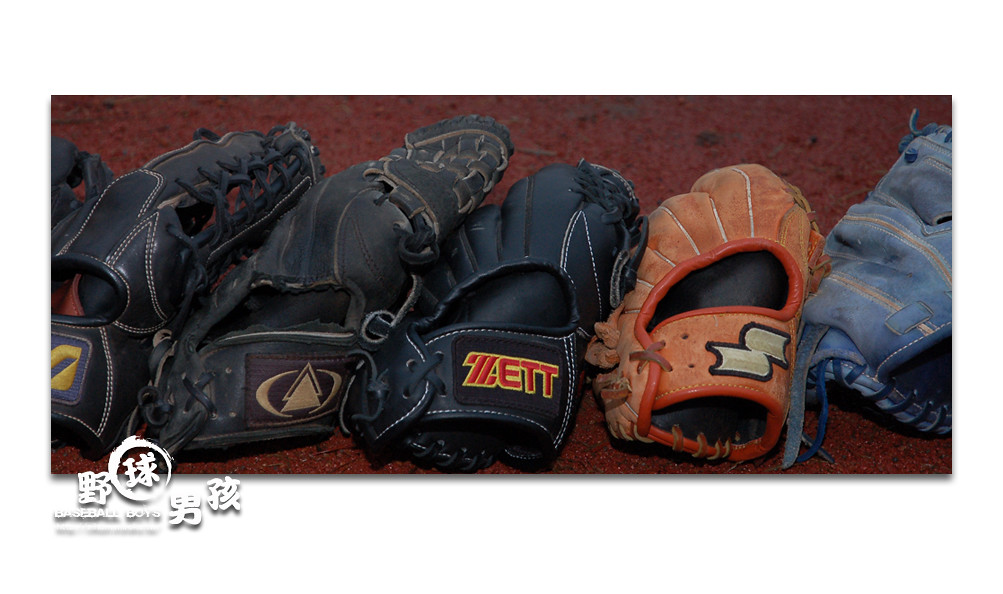This image features six baseball gloves lined up side-by-side on a painted red asphalt surface, resembling a dark brick color. From left to right, the gloves display a variety of colors and conditions. The far left glove is partially visible. The next glove is black and gold, followed by another black glove with a tan accent. The fourth glove is black with the word "ZETT" written in red and gold. Continuing right, the fifth glove is an orange leather with a white and black insignia on the wrist strap. The final glove, only partially visible, appears to be made of blue and tan material with white pinstripes. The gloves range from worn and distressed to newer and less used. In the lower left corner of the image, there is a logo with Japanese lettering, suggesting the image might be an advertisement for a baseball equipment manufacturer.